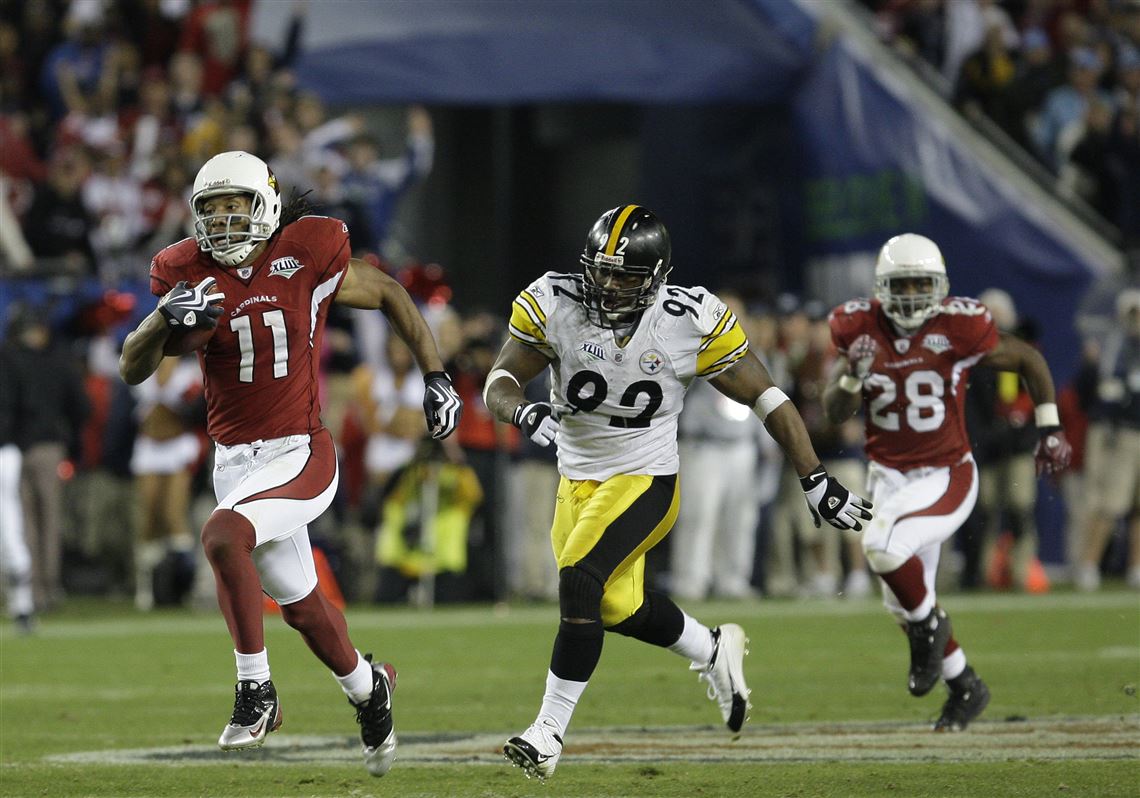In this vibrant action shot of an American football game, three players burst across a lush green field under the watchful eyes of a blurred crowd filled with enthusiastic fans and cheerleaders. The focal point is a player from the St. Louis Cardinals, donning a white helmet with a visible Cardinal logo, a maroon jersey bearing the number 11, matching maroon and white pants, white socks, and black and silver Nike cleats. This player clutches the football tightly in his right hand as he dashes forward. Trailing closely behind is a determined player from the Pittsburgh Steelers, wearing a distinctive black helmet with a yellow stripe, a white jersey with yellow accents on the sleeves, and yellow and black pants, emblazoned with the number 92. Further back is another Cardinal, number 28, dressed similarly to his teammate in maroon and white. The backdrop shows partially visible cheerleaders in white boots on the field and a sea of waving fans in the stadium seats. A blue awning hovers near the top of the image, framing the lively and dynamic scene.